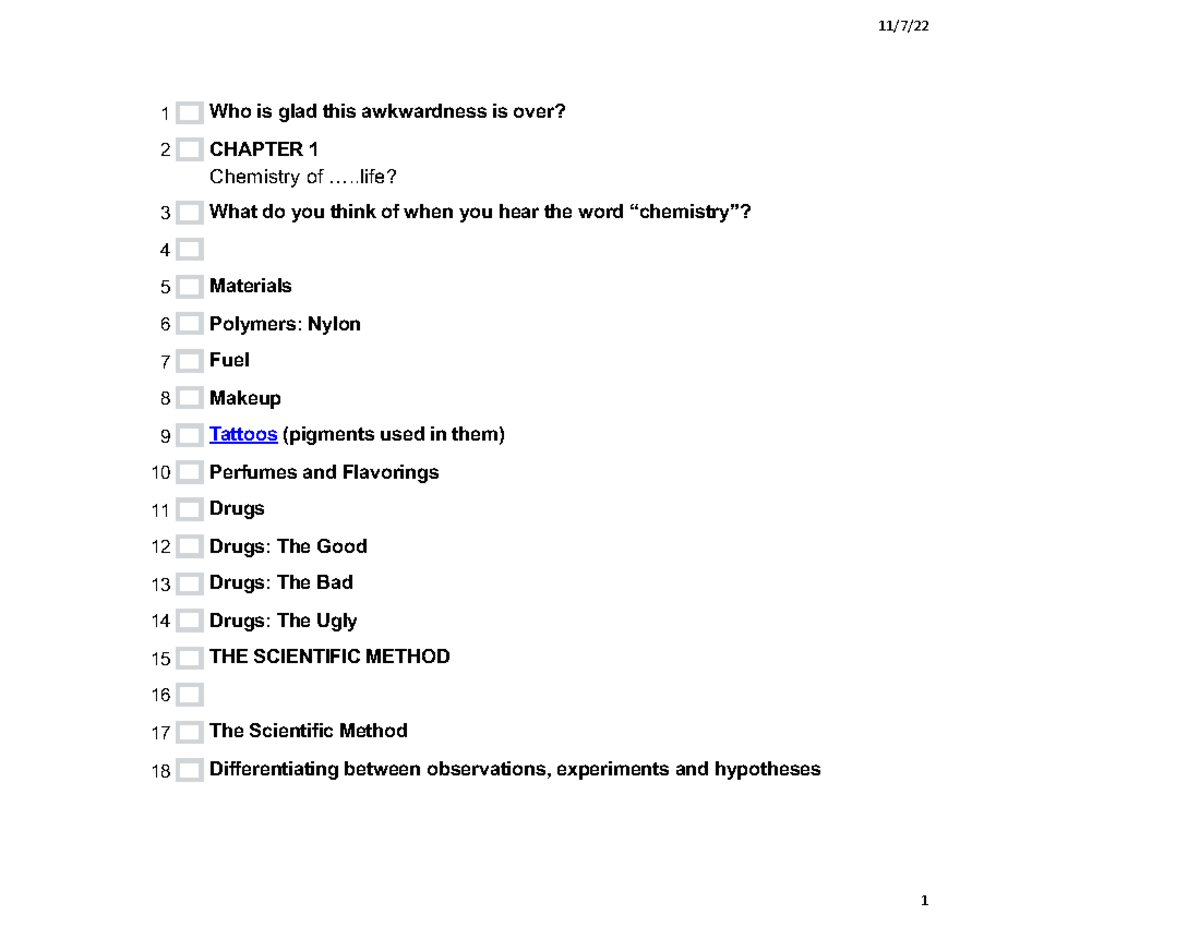On a white background, there appears to be a printed document resembling a detailed to-do checklist. The list is sequentially numbered, beginning at the top left with 1 and extending down to 18 at the bottom. To the right of each number is a gray, empty checkbox. Next to each checkbox is a line of text providing specific information, with each item occupying a single line. Here's the breakdown:

1. "Who is glad this awkwardness is over?"
2. "Chapter 1: Chemistry of Life"
3. "What do you think of when you hear the words chemistry?"
4. (This line is blank)
5. "Materials"
6. "Polymers: Nylon"
7. "Fuel"
8. "Makeup"
9. "Tattoos: Pigments used in them" (Note: "Tattoos" is hyperlinked and appears in blue)
10. "Perfumes and Flavorings"
11. "Drugs"
12. "Drugs: The Good"
13. "Drugs: The Bad"
14. "Drugs: The Ugly"
15. "The Scientific Method"
16. (This line is blank)
17. "The Scientific Method"
18. "Differentiating between Observations, Experiments, and Hypothesis"

At the very bottom center of the document, there is a large, prominent number "1." Additionally, at the center top of the document, the date "11 7 22" is printed, suggesting the date when the checklist was created or last modified.